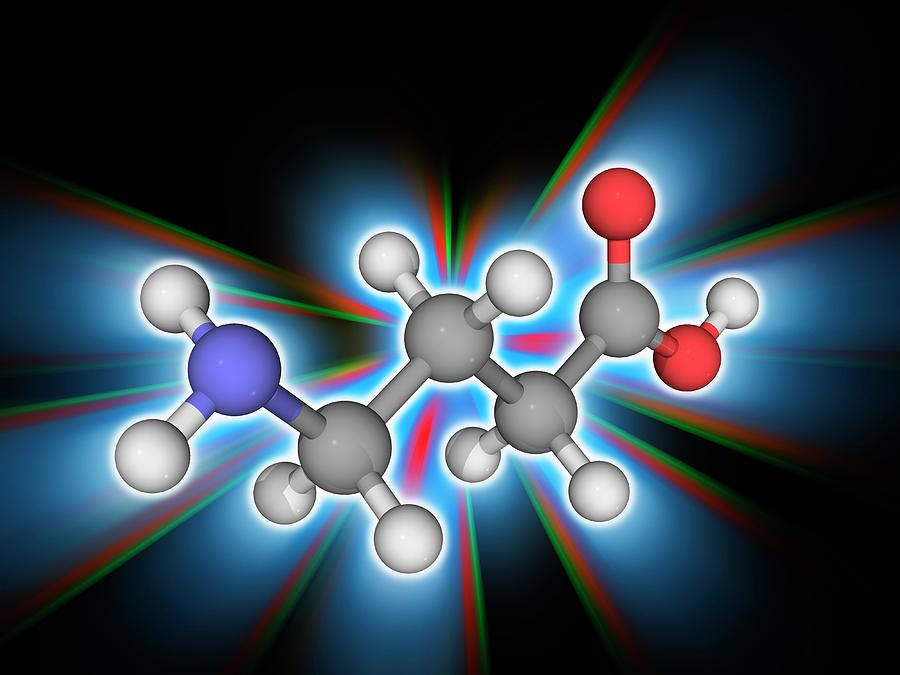This highly detailed computer-rendered illustration depicts a complex molecular structure set against a black backdrop. The central focus is a compound composed of several interconnected spheres, detailed with a radiant halo and multicolored light refractions. The compound features a prominent blue orb on the left side, extending from which are two nodules connected by a gray sphere. These gray nodules are central, each connected to additional spheres including red and white nodules. Specifically, the structure includes five primary spheres with intricate tubes fanning out into additional gray, white, and red spheres. Around the perimeter, nine smaller white orbs are distributed. Behind the molecular model, a soft white glow enhances the image, complemented by blue, green, and red rays of light that emanate from various points of the structure.